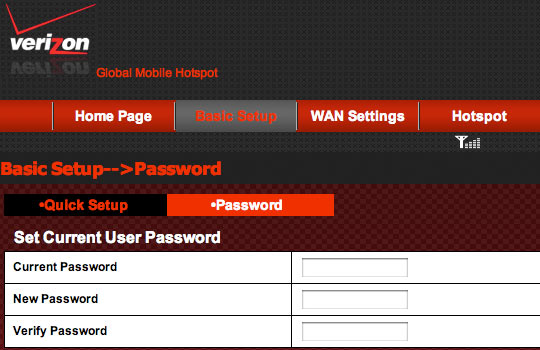This image is a computer graphic depicting the password setup page on a Verizon Global Mobile Hotspot website. It features a black rectangular background with a prominent Verizon logo in the top left corner, showcasing the company's name in white text with a distinctive red 'Z' and a red checkmark above the 'V'. Beneath the logo, "Global Mobile Hotspot" is written in red.

The main interface is divided into sections. At the top is a navigation bar with labeled buttons: "Homepage" (white on red), "Basic Setup" (grayed out with red text, indicating the current page), "WAN Settings" (white on red), and "Hotspot" (white on red). Below the navigation bar, there is a graphical element representing a tower, symbolizing the hotspot functionality.

The central focus of the page is the Basic Setup section, specifically for password configuration. Here, instructions in red text on a black background guide the user through setting up their password. The steps are clearly laid out with labels for "Current Password," "New Password," and "Verify Password," each accompanied by white text on black input fields where the user can enter the respective passwords.

In summary, the image effectively showcases the process for setting up a password on a Verizon Global Mobile Hotspot, emphasizing the clearly organized input fields and navigational structure.